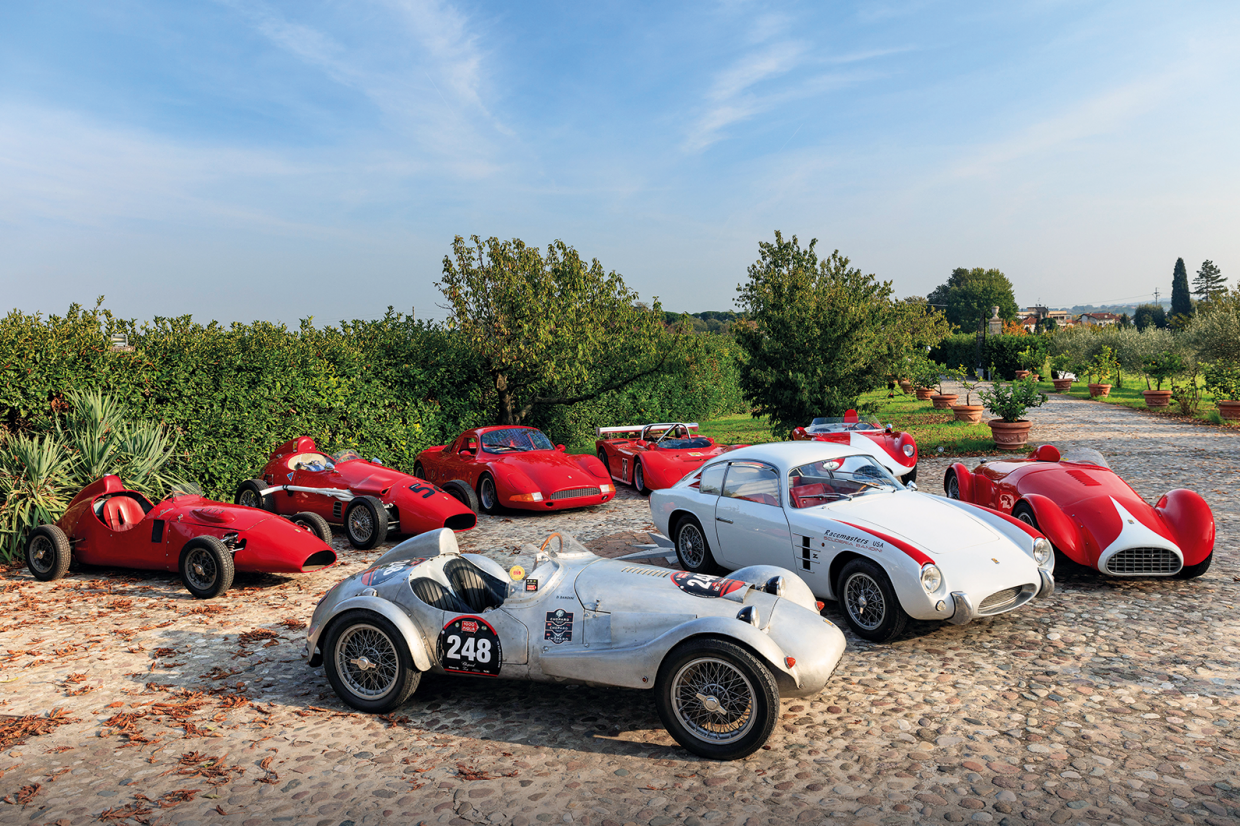This daytime, outdoor image, possibly taken in a European countryside, features a vibrant blue sky with light clouds and an expansive background of lower hills and green trees. The right side of the image displays buildings with distinctive orange rust-colored roofs and white walls, situated near a lush field and various bushes. The paved driveway, lined with potted plants and trees, bisects the image, leading into a collection of about nine cars. Among these, several are noteworthy: six red race cars, two white cars, and a silver car. Notable models include potential racing cars, with one bearing the number "248," a custom-made roadster, a vehicle resembling a Lamborghini, and another akin to a Porsche. The visual vibrancy of the scene is amplified by the greenery and natural elements surrounding the driveway.